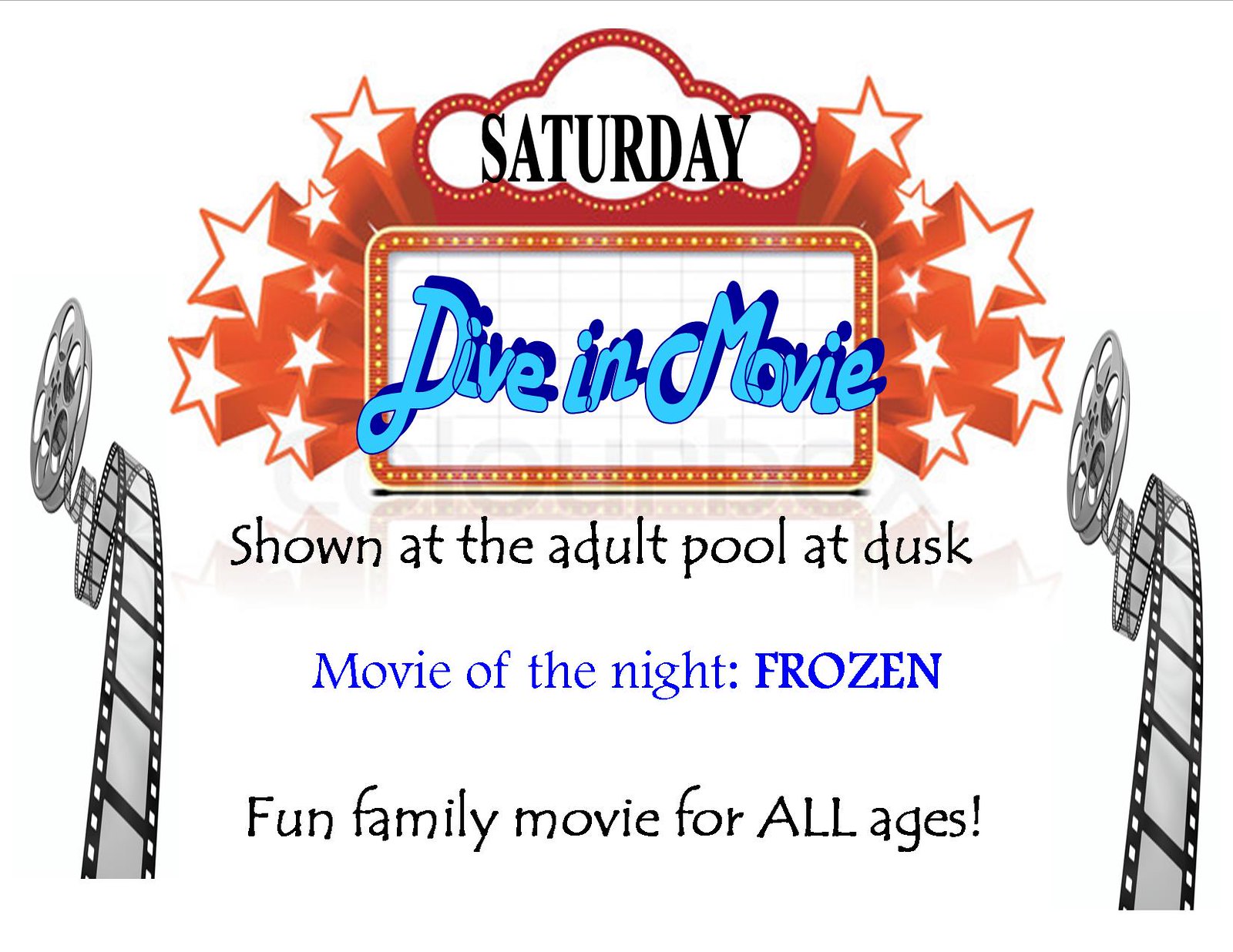The flyer for the "Dive-in Movie" event features an amateur-looking design that seems to be created using basic software, likely PowerPoint or Microsoft Word. The background is entirely white, overlaid with orange stars shooting out with motion trails. At the top, there is a white cloud-like graphic outlined with a wavy red striping and small yellow lights reminiscent of a classic movie marquee. Inside this cloud graphic, in black sans-serif font, it reads "Saturday."

Below this, a white rectangular box with rounded edges and an orange trim adorned with more yellow marquee-style lights contains blue text shadowed in dark blue that reads "Dive-in Movie." Flanking either side of the graphic are clipart-style metal movie reels with film strips cascading downwards.

The flyer further details the event with the text: "Shown at the adult pool at dusk. Movie of the night: Frozen. Fun family movie for all ages." Despite its unprofessional appearance and closely packed text, the flyer communicates the essential information about the family-friendly dive-in movie night.